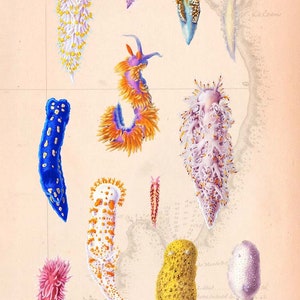The image is a detailed illustration of various colorful, worm-like microorganisms or caterpillars on a peach to light pink background. Each organism boasts a unique color palette and distinctive features. The center showcases a fuzzy bright orange caterpillar with blue antennae and a blue belly. To its left, a vibrant blue organism adorned with yellow dots stands out. On the right, a purple and cream-colored caterpillar appears feathery, while at the bottom, there's a white caterpillar accented with orange. Other notable creatures include a blue one with white spots, a curly blue one resembling a seahorse with black and blue protrusions, a yellow one speckled with black dots, and a white one with gold tips. Several organisms have spiky protrusions and intricate patterns of dots and stripes, adding to the image's overall vibrancy and uniqueness. The background ties them together, making it look like these colorful entities are moving upward or populating a shared space. There is no text to explain the image, leaving the viewer to marvel at the intricate and cheery designs.